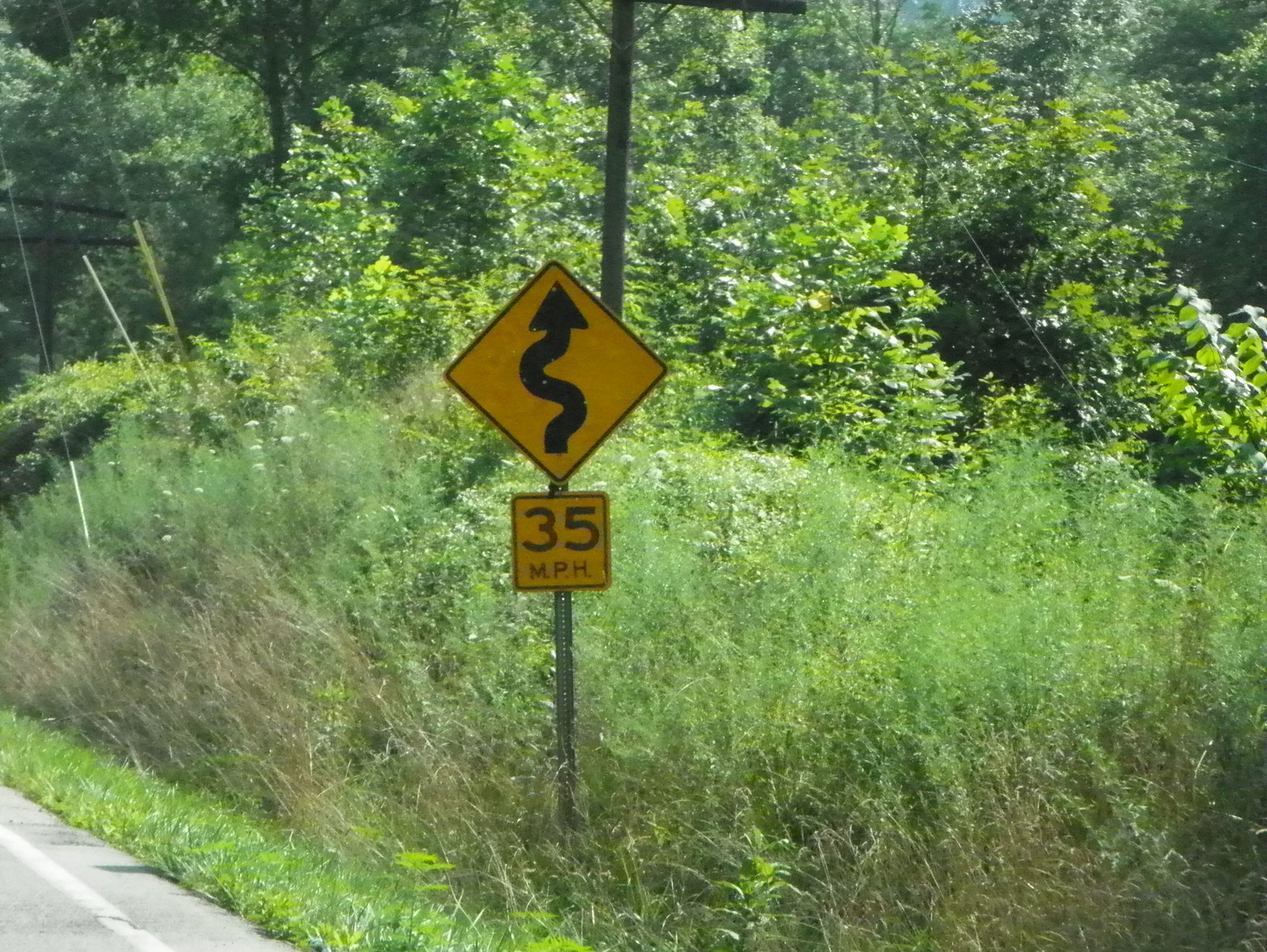This captivating image depicts a rural setting dominated by lush greenery, including tall grass, overgrown weeds, and a dense forest backdrop, suggesting an untamed, natural environment. A prominent feature in the foreground is a pair of road signs mounted on a metal post, signaling to drivers the conditions ahead. The upper sign is a vivid yellow, diamond-shaped traffic warning sign, featuring a bold black arrow that swerves to indicate a winding road. Below it, a slightly rounded square sign states the speed limit of 35 MPH in black letters. A glimpse of the cement road with a visible white stripe can be seen in the lower left corner, hinting at its proximity. The sunlight casts a clear, bright light over the scene, affirming it's daytime.